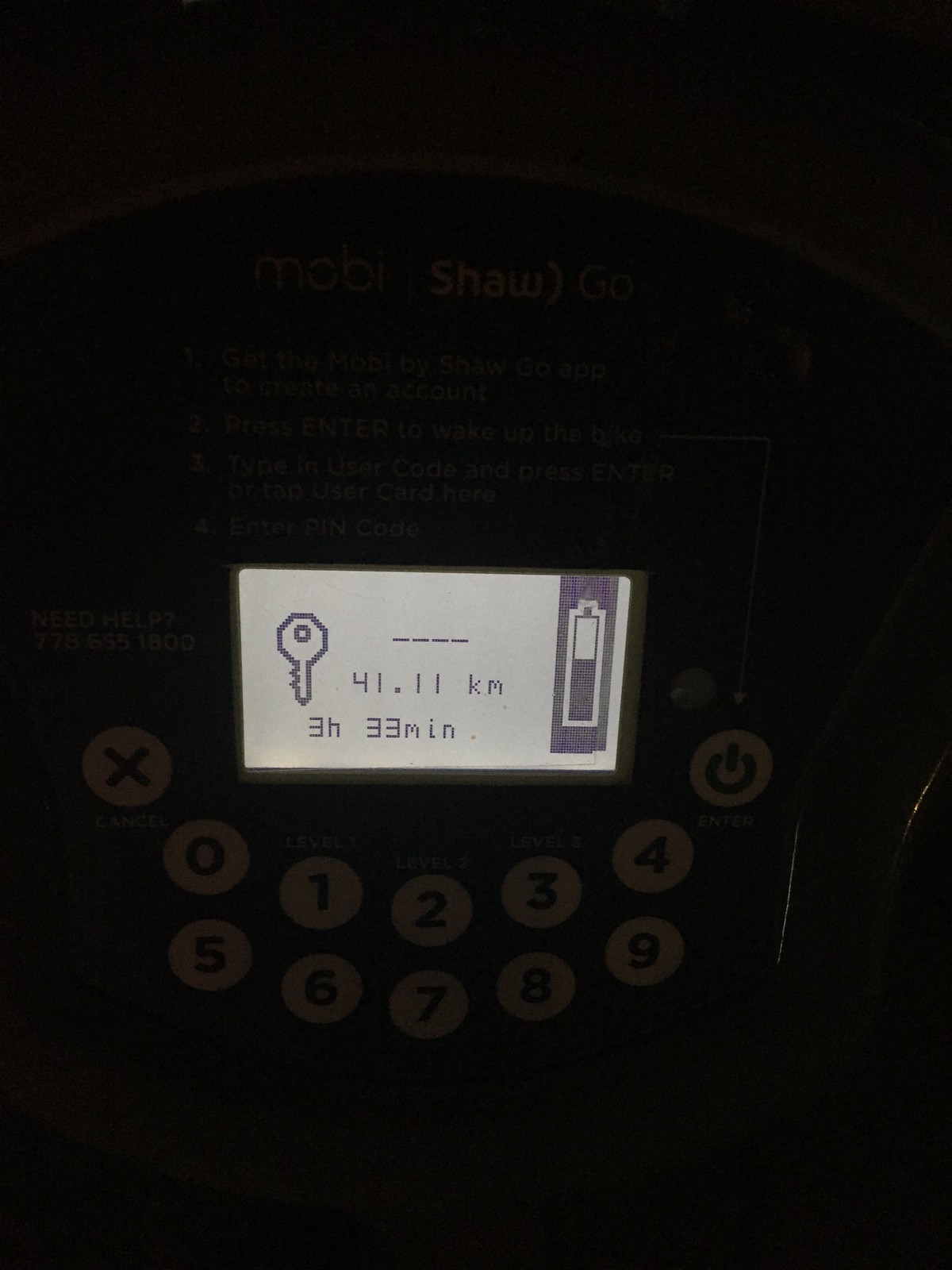The image depicts a dimly lit photograph of an electronic dashboard, possibly from an electric vehicle or e-bike. Dominating the scene is a small LED screen displaying various details: a key icon, a half-charged battery icon, and the figures "3 hours and 33 minutes" alongside "41.11 kilometers." Above the screen, "Moby Shaw Go" is faintly visible, indicating the system's name. It prompts the user to enter a pin code or tap a user card, with instructions like "Enter to wake up" and "Type in user code, then press enter." Below the screen, there's a numeric keypad with circular buttons numbered 0-9, an 'X' button on the left, and an 'On' button on the right. The entire background is enveloped in darkness, hinting that the photo might have been taken in low light using a cell phone.